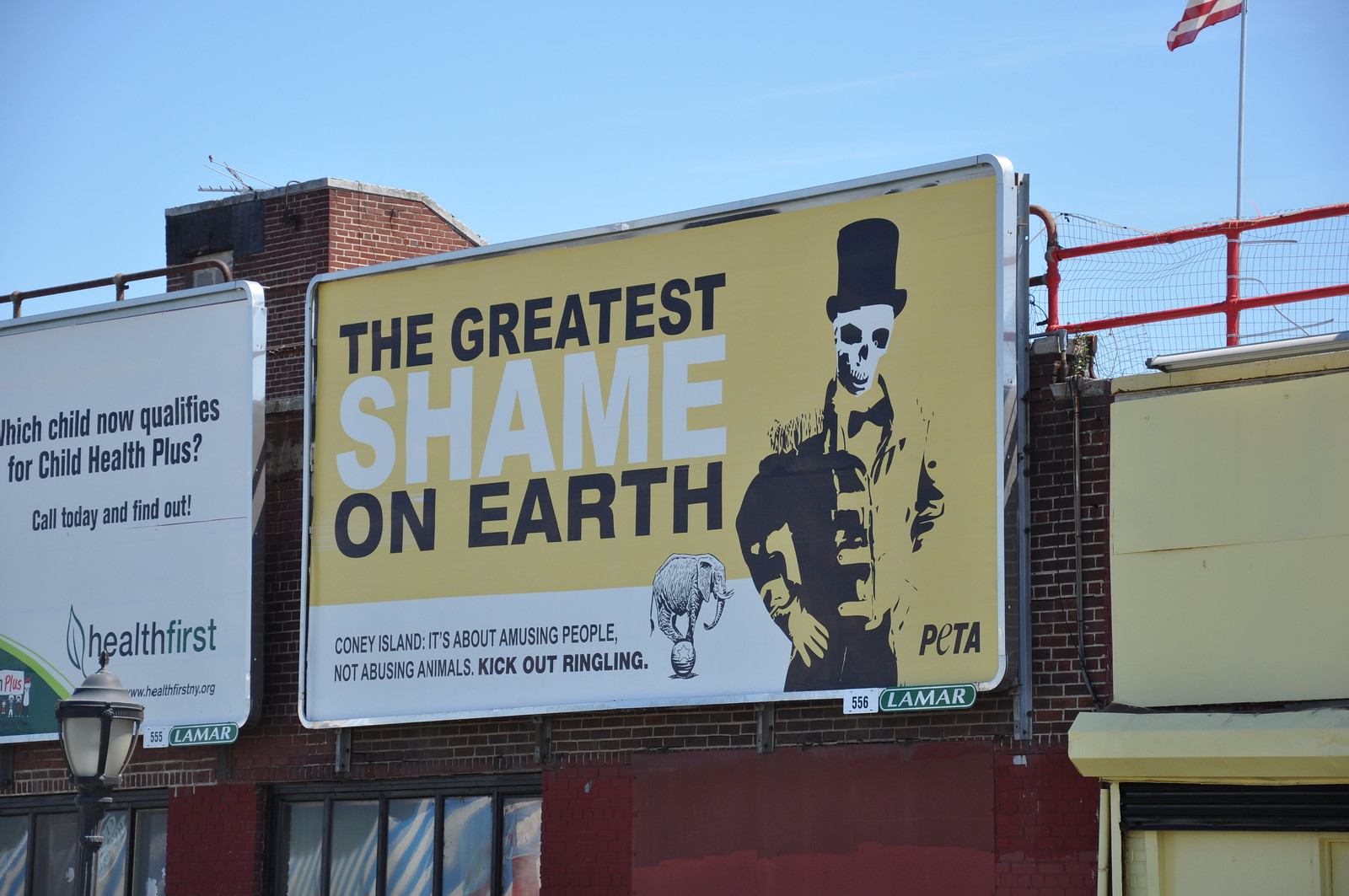The image features two billboards mounted on the walls of adjacent buildings. The billboard on the left, partially obscured, is predominantly white with the words "Health First" in the lower right corner, suggesting a health insurance advertisement. The billboard on the right, clearly visible, is brightly colored in yellow and features a skeleton dressed in a tuxedo and black top hat in the right corner. Above the skeleton, bold black text reads "The Greatest," followed by smaller white text stating "Shame" and black text underneath it saying "On Earth." Inside a white box at the bottom, black text reads "Coney Island." Below, it further states, "It's about amusing people, not abusing animals. Check out Ringling," accompanied by an image of an elephant. The lower right corner of this billboard bears the acronym "PETA" in black letters. Both billboards are wide rectangular shapes, approximately 15 feet wide by 10 feet high. The setting appears to be in Coney Island, judging by the mention of local shops and the context provided in the billboards.